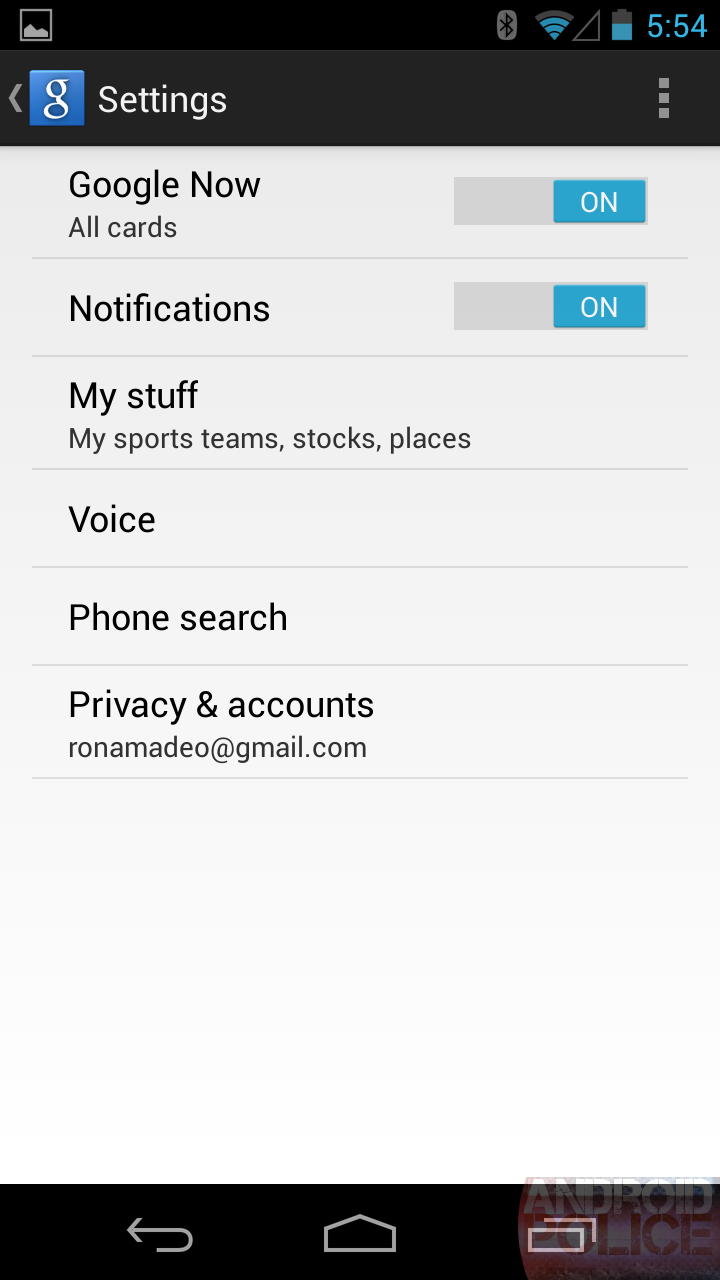This is a detailed screenshot capturing a section of a mobile device screen from an application, likely a settings or system info tab. At the top of the image, there is a black status bar that includes several icons: a gray Bluetooth symbol, a blue and gray Wi-Fi signal icon, a triangular symbol, and a light blue battery icon which indicates the time as 5:54.

Moving down, there is a thin gray tab featuring a centered blue and white ‘G’ for Google, labeled "Settings." Next to this tab are three horizontal lines and three vertical dots, both in gray, indicating a menu or additional settings.

The main content area has a gray background and black text. This section details the configuration and options available for Google services. There are gray boxes with blue squares labeled "Google Cards Now," "Google Now all cards on," and "Notifications on." Below this, additional information highlights various settings categories like "My Stuff," "My Sports Team," "Stocks," "Places," "Voice," "Phone Search," "Privacy," and "Accounts." The email address associated with these settings is clearly shown as grownmade@gmail.com.

At the bottom of the screenshot, there is a black navigation bar. It includes three white icons: a back arrow, a home icon, and a recent apps icon represented by two layered squares.

Overlaying the image appears to be a faint watermark—"Android Police"—with the word "Android" in white and "Police" in red, accompanied by a red circle. Faint gray lines run between each of the words for further separation.